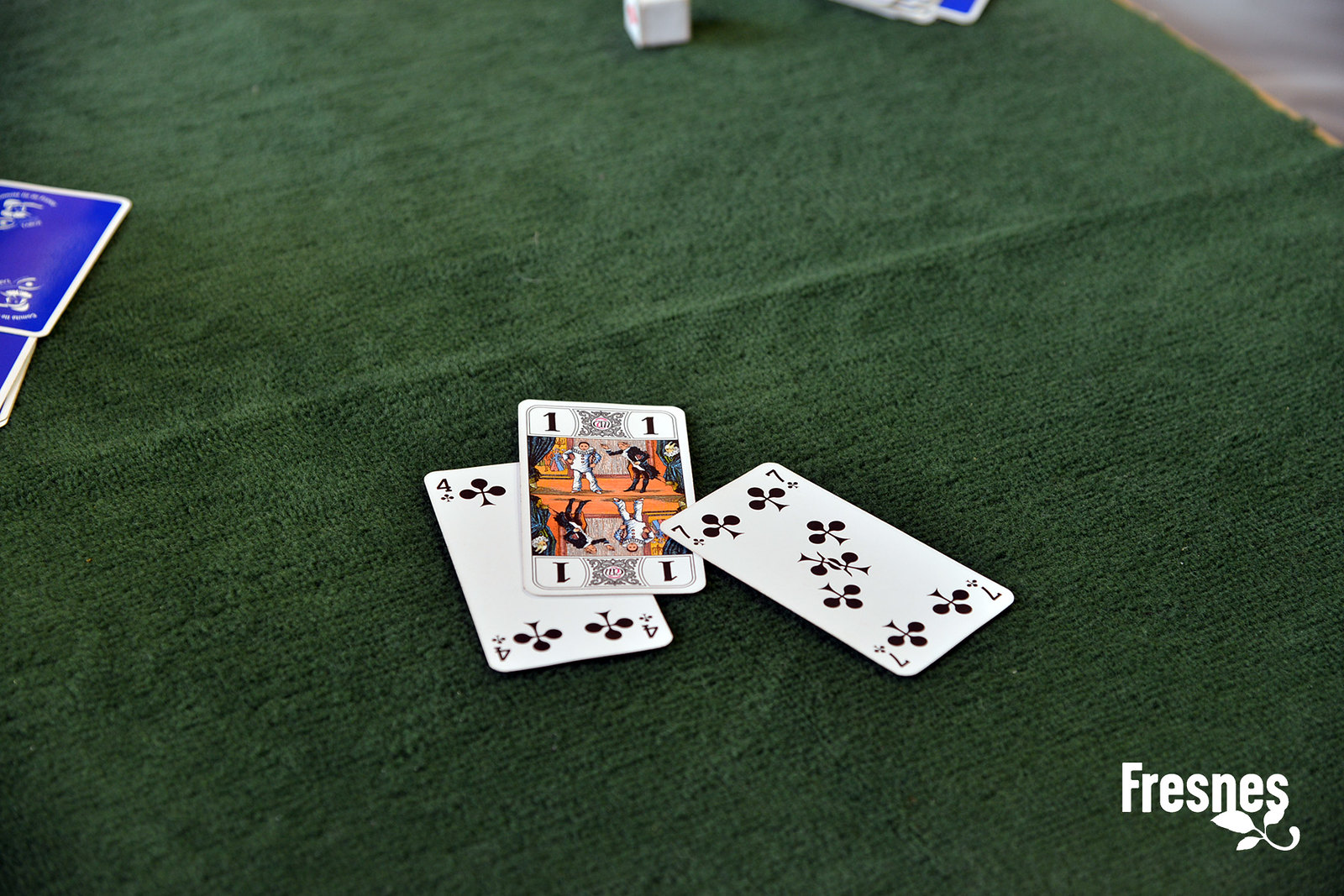In the image captured with a standard camera, a card game is in full swing on what appears to be a green, grassy-looking basement carpet. Alternatively, it could be a tablecloth, but it resembles the texture of basement carpeting. The central focus of the image is on the cards laid out for the player positioned towards the middle to the lower section of the frame. This player has three cards turned face-up: a Four of Clubs, an Ace of Clubs, and a Seven of Clubs. To the right side of the image, three more cards lie face-down, displaying only their blue backs. Additionally, at the top of the picture, the tiny corners of a couple of blue-backed cards peek into view. Towards the middle top of the image, a cube that resembles a dice is placed, but it lacks markings on one side, raising questions about its purpose. Finally, at the bottom of the picture is the word "FRESHNESS," written in capital letters with a stylized white leaf curling up in one corner, adding an intriguing element to the scene.